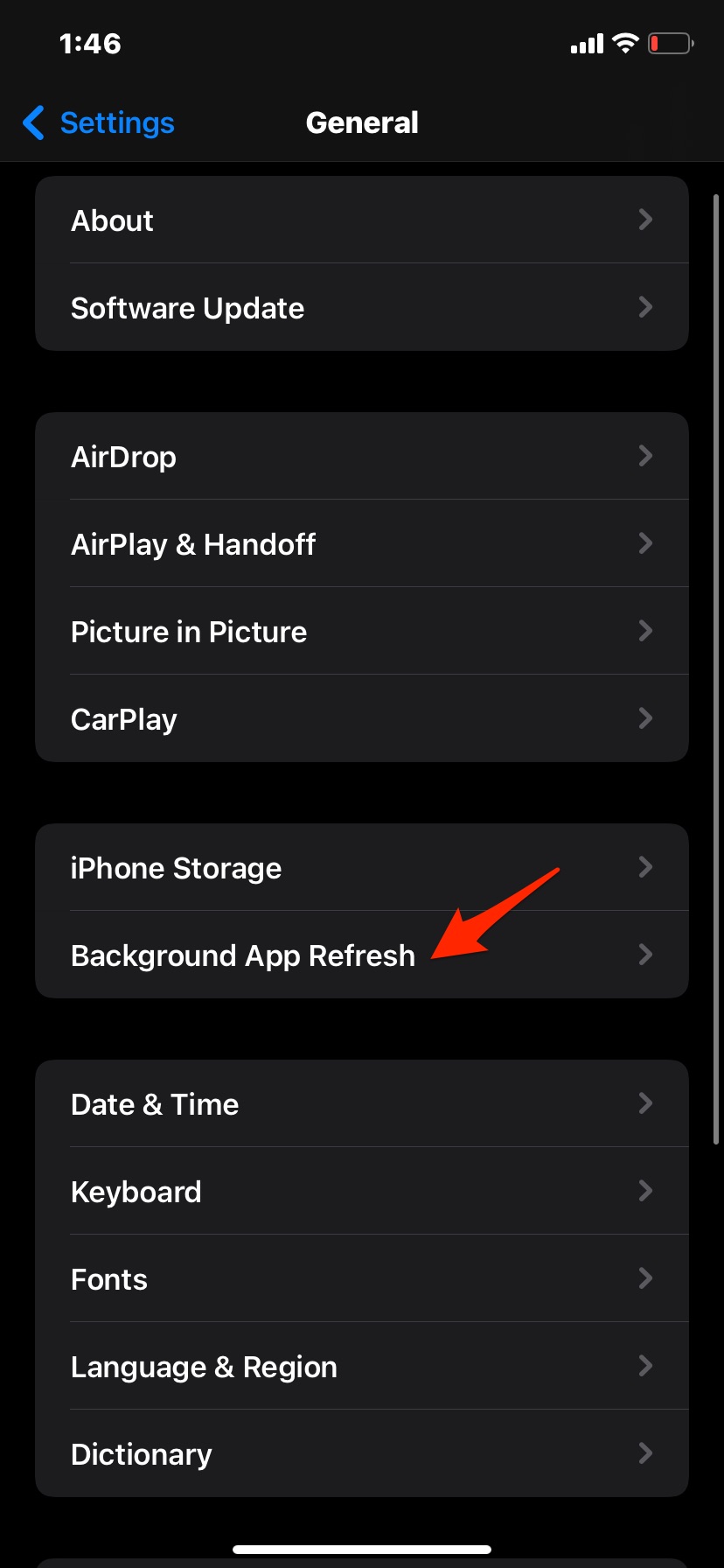This image is a screenshot of an iPhone's "Settings" menu under "General." The background of the screen is black, which contrasts with the blue-highlighted "Settings" title at the top. The general text throughout the menu appears in white for clearer readability. The status bar at the top of the screen shows the time as 1:46 and indicates a full cellular signal.

Below the "General" heading, the menu lists several options each with a rightward-pointing arrow, indicating they are clickable for more details. Starting with:

1. **About**
2. **Software Update**

These are followed by groupings of settings, including:

- **AirDrop**
- **AirPlay & Handoff**
- **Picture-in-Picture**
- **CarPlay**

Further down, we find:

- **iPhone Storage**
- **Background App Refresh**

A prominent red arrow in the screenshot specifically points to "Background App Refresh," drawing attention to this option.

The final section of the menu includes:

- **Date & Time**
- **Keyboard**
- **Fonts**
- **Language & Region**
- **Dictionary**

The screenshot comprehensively covers all visible options within the "General" settings menu of an iPhone.